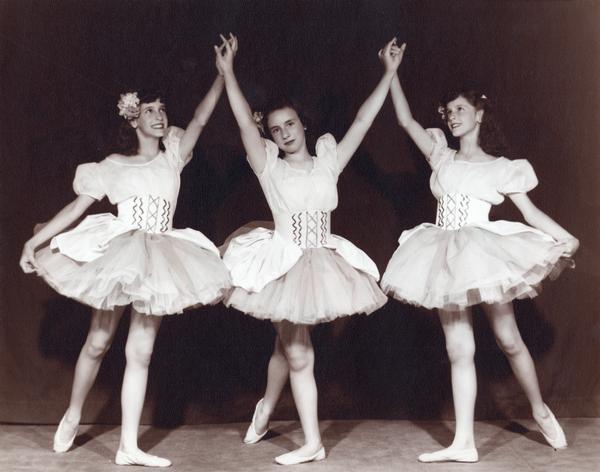This is a square, old, black and white photograph, set indoors against a dark black curtain that stops just shy of touching the stage floor, leaving a small gap visible at the bottom. It captures three young Caucasian women, possibly early to mid-teens, standing side by side in ballerina costumes, which include white tutus with corsets, sashes, and ballerina shoes. The women have their hair adorned with bows, adding to the old-timey aesthetic of the image, which shows signs of fading around the edges. The central figure stands in a classic ballet pose, with one foot pointed behind her and the other turned, her arms gracefully outstretched above her head while holding the hands of the two women beside her. These two women have similarly one leg extended back and one arm raised, each clasping the hand of the central figure, collectively forming an 'M' shape. Their expressions suggest that they are either about to perform a dance routine or practicing, radiating a sense of happiness and joy derived from their activity.